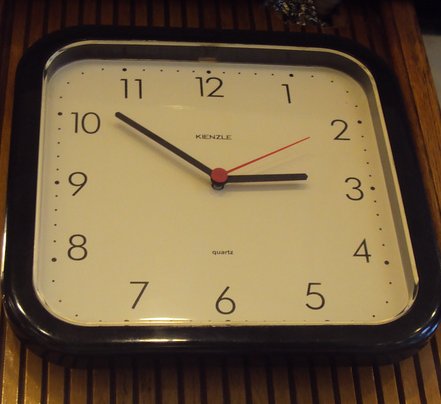This photograph features a close-up of a square wall clock with rounded corners. The clock boasts a black plastic housing surrounding an all-white face. Standard English numerals from 1 through 12 are arranged in a clockwise direction. The hour hand points just before the 3, the minute hand is slightly past the 10, indicating a time of approximately 2:52. The red second hand is aligned with the 2. At the top center of the clock, the brand name "Kenzel" is prominently displayed, while the bottom center features the word "Quartz," hinting at the clock's mechanism. The background reveals the clock is mounted on a brown wooden wall with vertical slats and visible gaps. The right edge of the image shows part of the wall, with an indistinct object partly visible behind it.